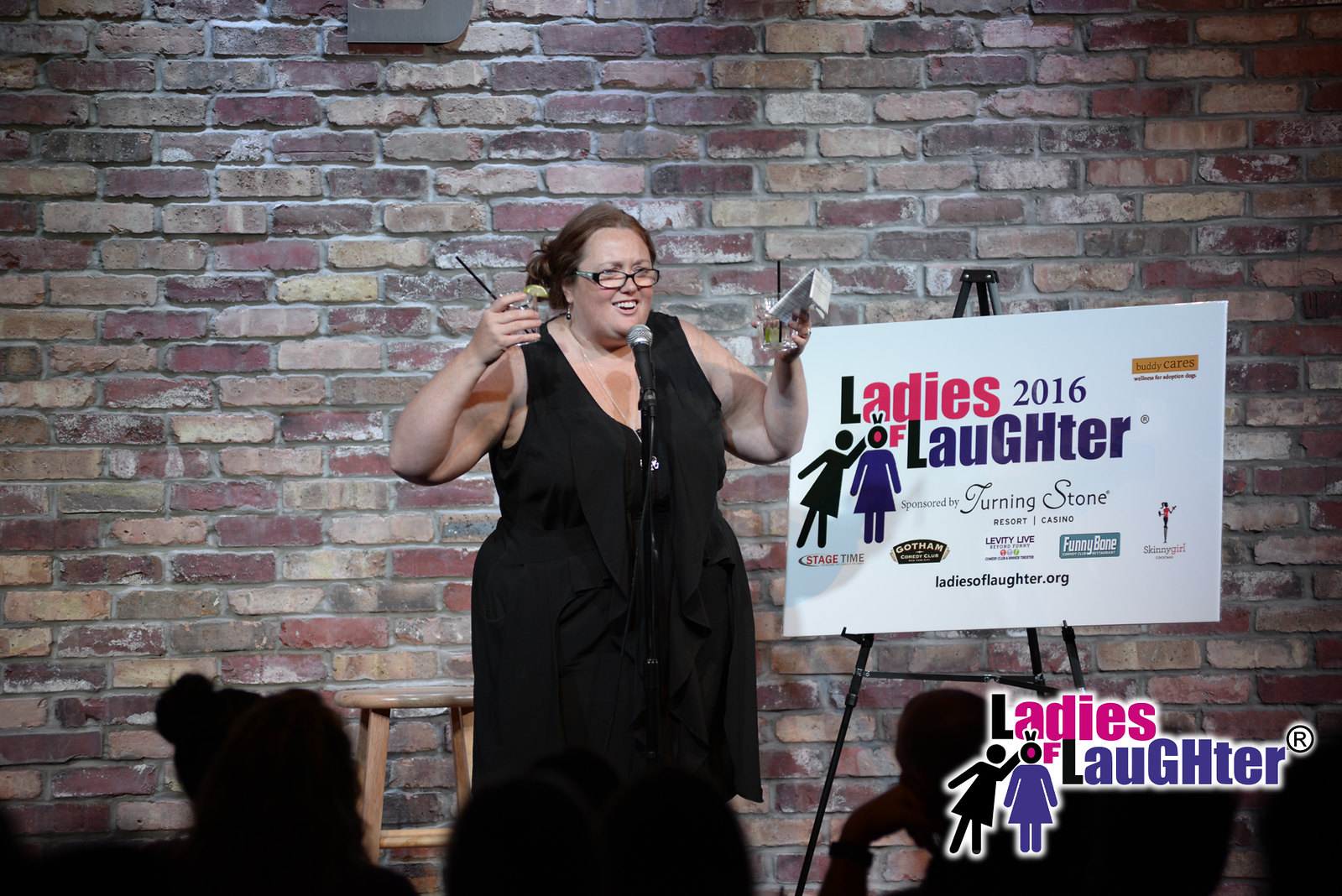In the photo from a 2016 "Ladies of Laughter" stand-up comedy event, a lively woman is captured mid-performance. She is standing in front of a traditional brick wall, indicative of many comedy club settings, and is energetically engaging with the audience, evident from her animated gestures. With a broad smile and glasses, she is dressed in a black dress and has her hair tied back in a bun. In her right hand, she holds a drink garnished with a lime and a large pink and black plastic straw, while her left hand holds another similar cup along with a piece of paper that could be her notes. She speaks into a microphone, and behind her, there is a wooden stool adding to the typical stand-up comedy ambiance. The background features a poster on a tripod, showcasing an emblem of women’s outlines and the text "Ladies of Laughter 2016" in pink, purple, and black. Various sponsors such as Gotham Comedy Club, Levity Live, Funny Bone, Skinny Girl, and Stage Time are listed, and the website ladiesoflaughter.org is also visible. The show is further branded with the "Ladies of Laughter" logo prominently placed in the bottom right corner of the image. Silhouettes of the audience can be seen, enhancing the live and intimate atmosphere of the comedy event.